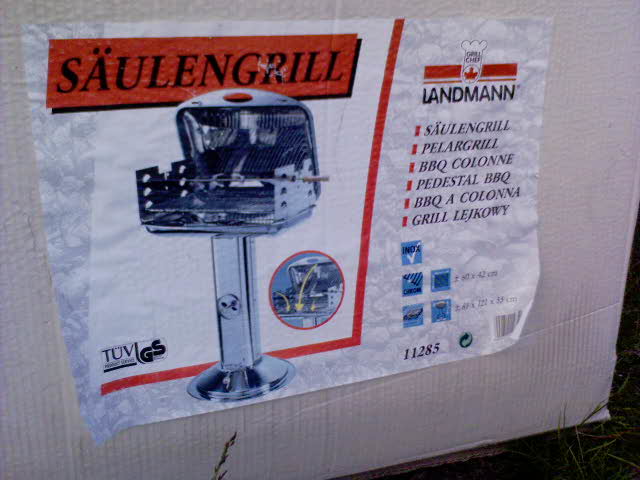This outdoor color photograph captures a slightly angled view of a label affixed to the side of a white box. The label is predominantly white and features an orange rectangle in the top portion, within which black capital letters spell out "S-A-U-L-E-N-G-R-I-L-L." Below this is a depiction of an open, standing grill made of stainless steel, with its front facing to the left. To the right of the grill image, there is another orange rectangle with a black outline of a chef's hat and the word "LANDMANN" (spelled with two 'N's) in bold black capital letters underneath.

Further down on the label, there are six bullet points in black capital letters. The points list different names and types of grills: "SALON GRILL," "PERLAR GRILL," "BBQ COLONE," "PEDESTAL BBQ," "BBQ A COLONA," and "GRILL LA GECANAO." The right corner of the label is partially peeled. At the very bottom of the label, a number "11285" is visible. The base appears to be a well-defined pedestal with a round base and a square column leading up to the grill, suggesting this grill might be designed for permanent installation. The background is a dark black color with some lighter scratches or lines, and the bottom part of the frame briefly shows the floor before it is cropped out.